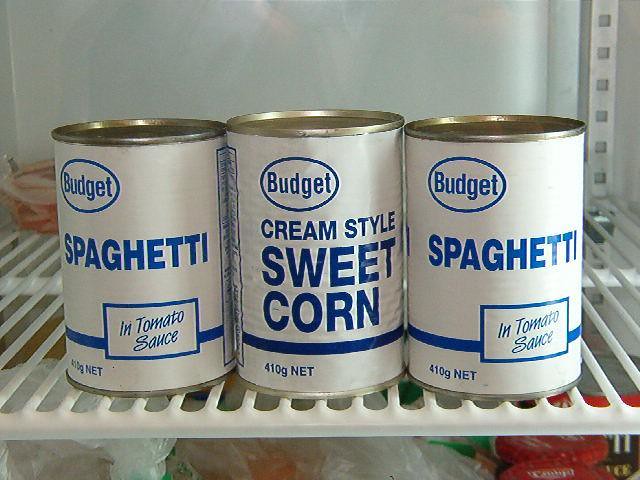The image features a close-up view of a shelf, potentially inside a refrigerator, captured at or near eye level. The background is a flat, white surface complemented by a grid of white wire bars running vertically and horizontally. Prominently displayed on the shelf are three cans, each with silver lids and white labels that read "budget." The cans are labeled as containing spaghetti, cream-style sweet corn, and another spaghetti. Towards the rear of the shelf, a distinct red object is visible, though its specifics are unclear. Below the cans, plastic bags containing what appear to be fruits or vegetables occupy the lower shelf space.